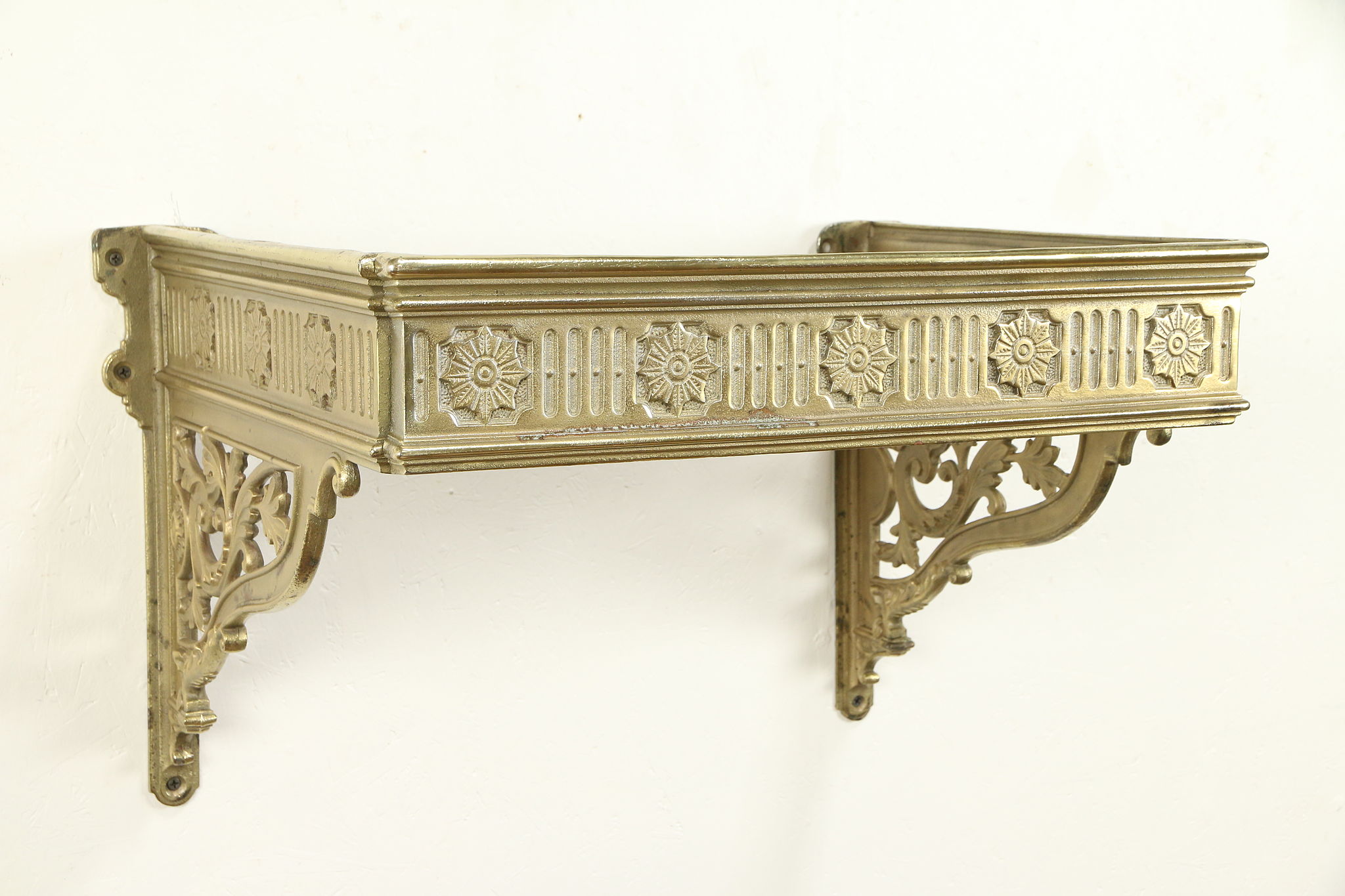The image shows an ornate, vintage-style shelf screwed into a white wall. Crafted in gold, the shelf includes a scrolling motif with a leaf design that extends from the lowest screw to the farthest part of the shelf, complemented by a worn, antique appearance. The front of the shelf features five floral decorations, while each side displays three more. The shelf itself is small with low raised sides, ensuring items placed on it won't easily fall off. Both sides are secured to the wall at the bottom with visible screws. The design includes intricate brackets beneath the shelf, adding to its decorative appeal.